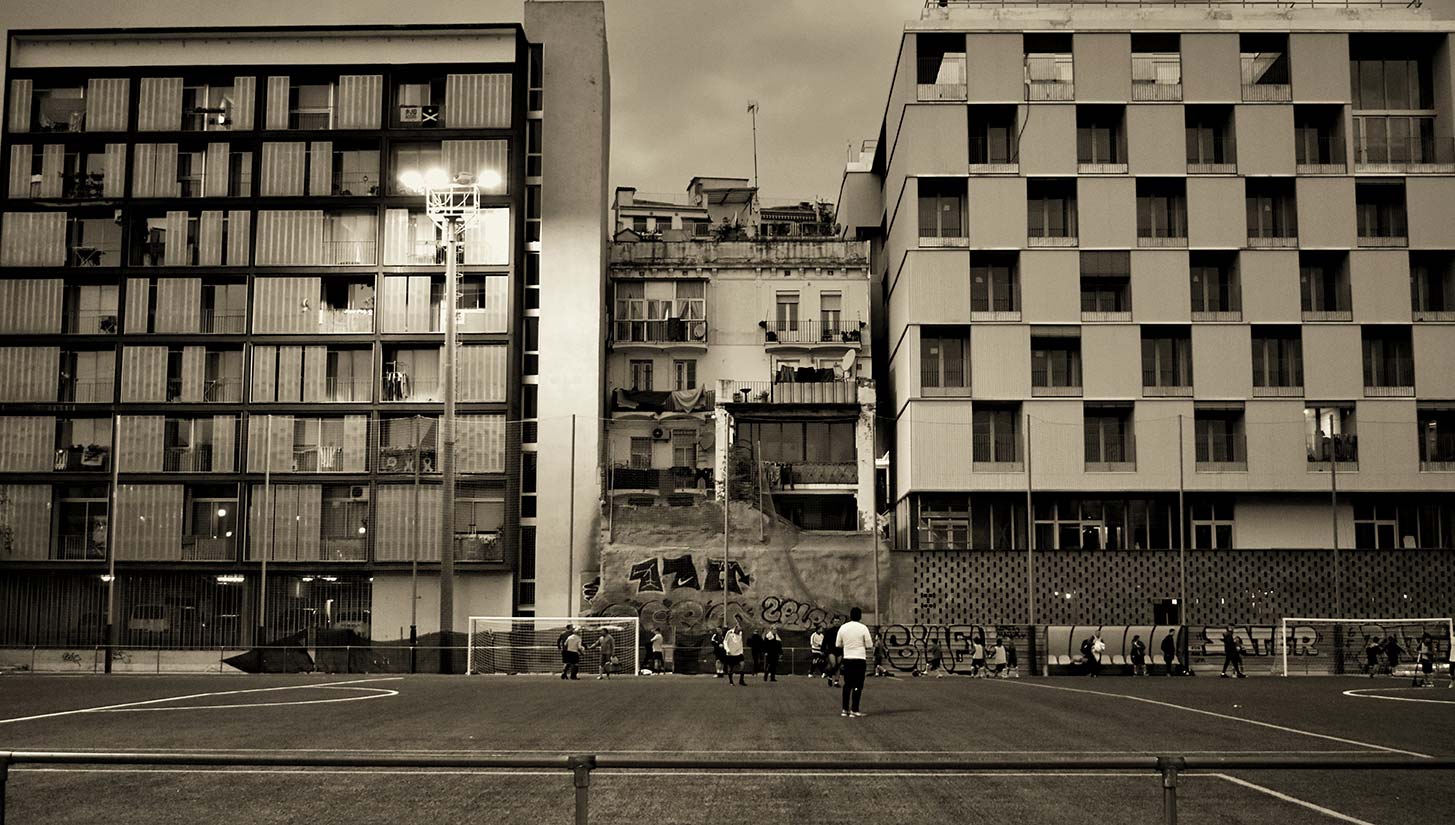This black-and-white photograph captures a nighttime scene in a city, focusing on a soccer field nestled between two large apartment buildings. The buildings, each rising four or five stories, are not luxurious but densely inhabited, possibly housing projects. The photo reveals a smaller, older building with terraces, positioned between the taller structures. The field itself, illuminated by tall stadium lights against a gray, cloudy sky, shows a group of people engaged in a casual soccer game, absent of uniforms, suggesting an informal, pickup match. The ground, marked with white lines and soccer goals, may also serve as a multi-use sports court. Graffiti adorns a concrete wall and a fence surrounding the field, adding urban texture to the scene. The overall image is slightly zoomed out, emphasizing the everyday life and gritty character of the urban environment.